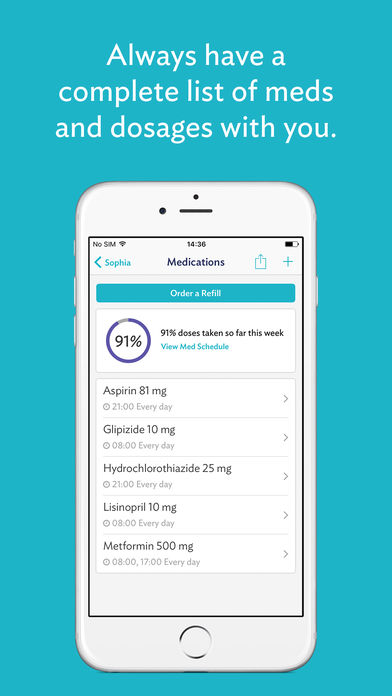Promotional image for a health-related app featuring a sleek, detailed interface: The photo displays a white iPhone with a built-in home button, against a serene turquoise-blue background. At the top in bold white text, it reads, "Always have a complete list of meds and dosages with you." The iPhone screen showcases the app's main interface. The app, titled "Medications," features a clean white background, with a prominent turquoise button labeled, "Order a refill." Below this are informative statistics: "91% doses taken so far this week" and a prompt, "Review med schedule." The interface further lists the user's medications, including aspirin, glyphosate, hydrochlorothiazide, lisinopril, and metformin, managed by a user named Sophia. The image, with its tall rectangular dimensions, effectively resembles a helpful and user-friendly app screenshot designed to ensure users maintain an organized and accessible medication schedule.